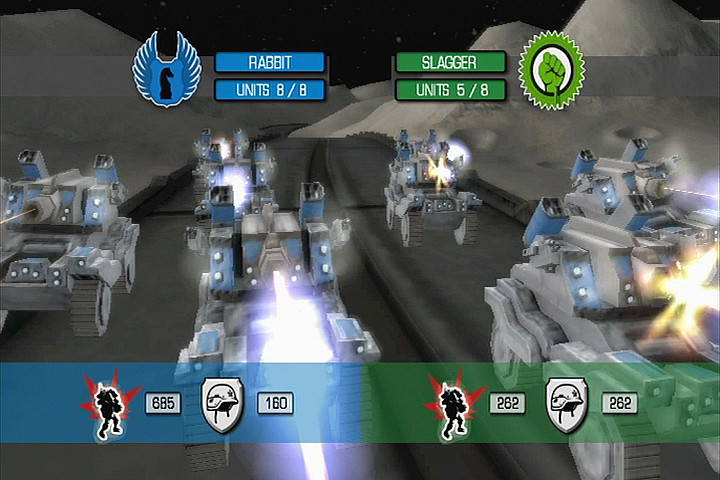The screenshot depicts a computer-generated image from a video game set on a moon-like landscape with grey, cratered ridges in the background. A black road cutting through the barren terrain is home to various blue and grey tanks equipped with turrets and rocket launchers, rolling on tires rather than treads. The tanks are moving towards the viewer and are engaged in what appears to be a battle.

At the top of the screen, two emblems signify opposing teams: on the left is the blue team symbolized by a knight chess piece with a winged background, captained by "Rabbit," who has a full complement of 8 out of 8 units remaining. On the right, the green team features a raised fist emblem within a circle and is led by "Slagger," who has 5 out of 8 units left. A dual-colored banner at the top transitions from blue to green, indicating the ongoing match between the teams.

A detailed status bar at the bottom of the screen shows additional metrics. For the blue team, an icon of a soldier reads "685" and a helmet symbol displays "160." Meanwhile, the green team is trailing with both soldier and helmet indicators showing "282." This comprehensive layout, complete with various numerical statistics and team symbols, suggests that the blue team is currently winning the engagement.